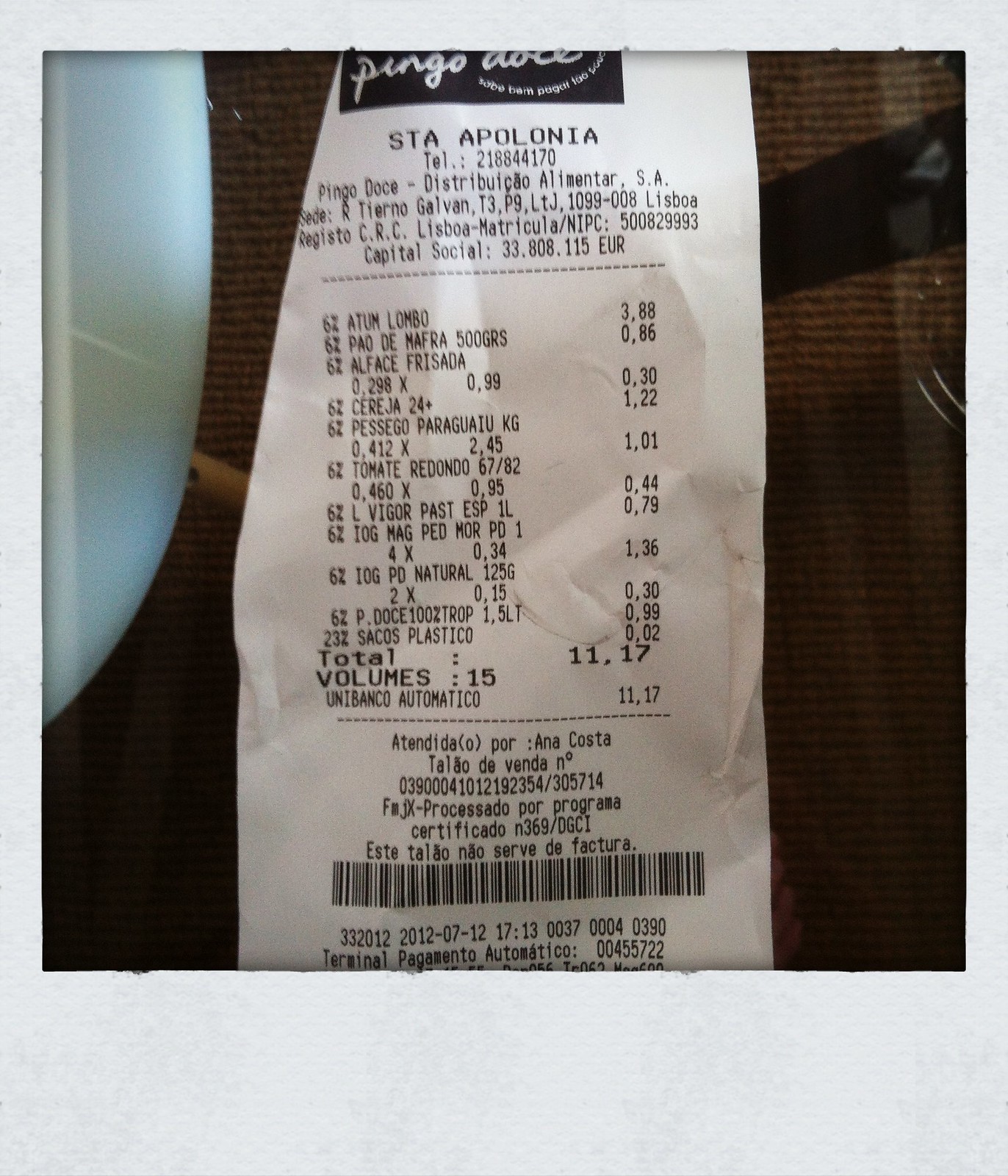This Polaroid photograph captures a receipt from a location named Apollonia, featuring the telephone number 218-844-170. The address on the receipt indicates that it is from an out-of-country establishment. The setting appears to be a restaurant, as suggested by the brown tablecloth in the background and a white bowl or plate placed next to the receipt. The receipt and its surrounding elements subtly hint at an international dining experience.